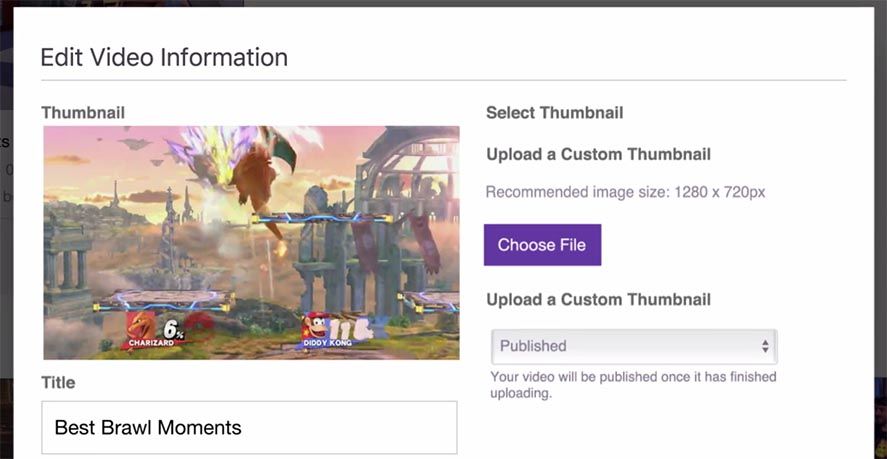The image depicts a website with a black border. The primary background color of the webpage is white. At the top in bold black letters, it reads "Edit Video Information." Below this, there is a thin gray horizontal line. The section following the line is labeled "Thumbnail" in black text, under which a vibrant and colorful image is displayed. The image appears to be a screenshot from a video game featuring cartoon-like graphics. The scene depicts what looks like a battlefield with several ruins and an explosion emanating multicolored sparks. Two characters from the game are engaged in combat, and their scores and player images are visible.

Below the thumbnail image, the page includes a label "Title" next to a white text box that contains the text "Best Brawl Moments." To the right of this text box, there are options labeled "Select Thumbnail" and "Upload a Custom Thumbnail," with a recommended image size of 1280 by 720 pixels. Further down, there's a prominent purple button labeled "Choose File" in white text, which is followed by another prompt to upload a custom thumbnail. Here, a light gray box is labeled "Published," featuring up and down arrows for selection. Lastly, there's a note in gray text stating, "Your video will be published once it has finished uploading."